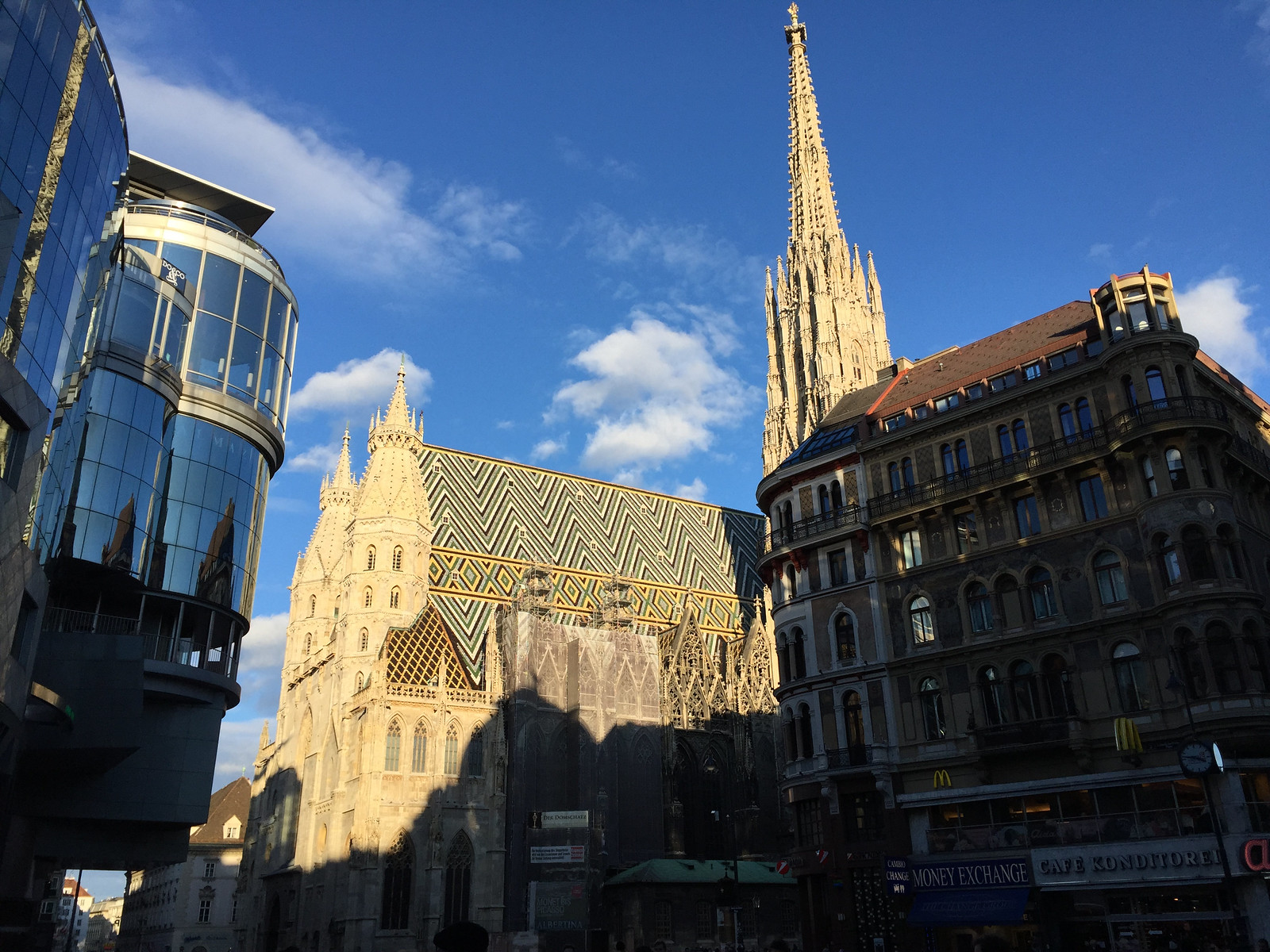This outdoor photo showcases a vivid scene under a bright blue sky with wispy clouds, seemingly taken in the early morning or late evening due to the long shadows. Dominating the center is a large, light tan medieval or gothic cathedral. Its defining feature is a tall, pointed gothic spire, accompanied by multiple smaller spires beneath it, contributing to the intricate design. The cathedral also sports a distinctive zigzag pattern on its roof. To its left, there's a modern-looking building with a rounded, glass facade that gleams in the sunlight, juxtaposing the historical architecture with contemporary style. The base of the image is engulfed in shadow, making some details obscure, including a darker, possibly brown building on the right that might serve as apartments or a hotel, exuding a European charm.